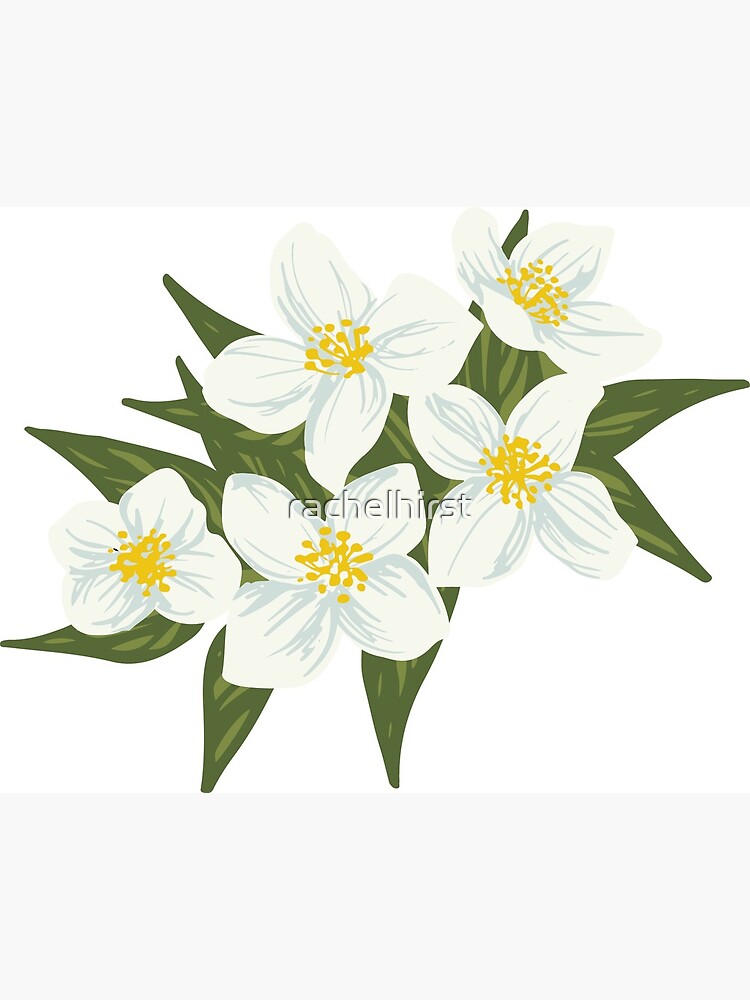This is a computer-generated image titled "Rachel Hurst" featuring five white flowers, possibly lotus blossoms or white poinsettias, with multicolored green leaves. The composition is viewed from a top-down perspective, creating a flat, 2D effect in a graphic art style. The flowers are adorned with olive green and gold accents, and their white petals and yellow stamen stand out sharply, contributing to a calming visual presence. Despite the lack of a discernible background, the arrangement's simplicity and precise detail evoke a sense of peace and beauty.